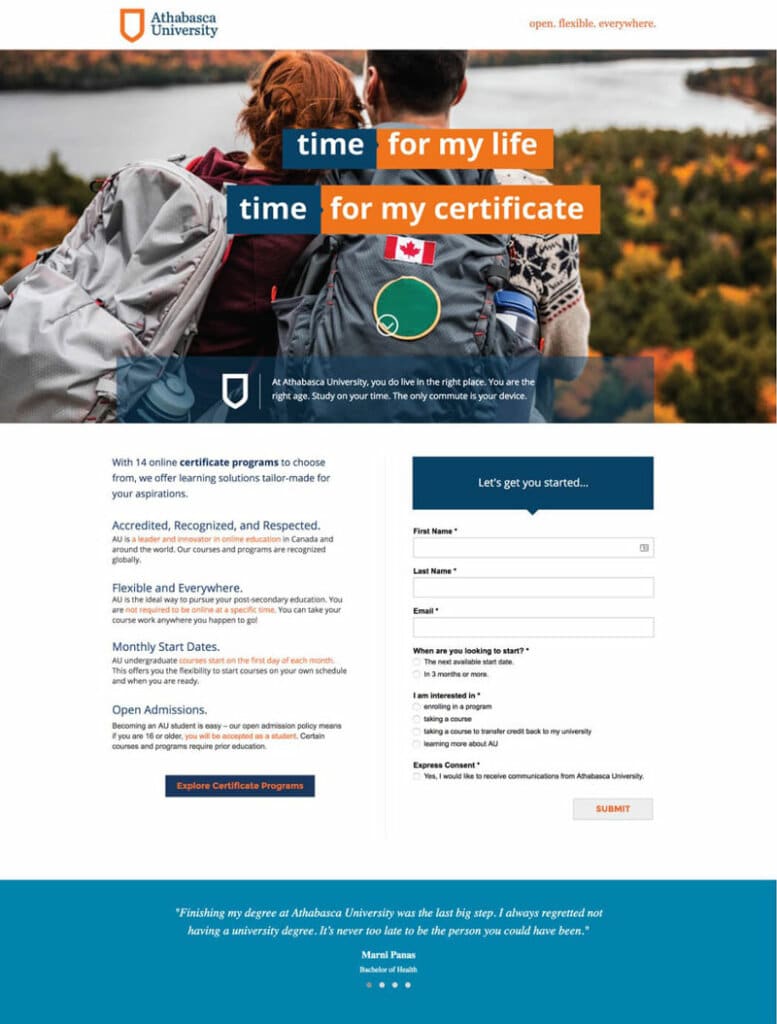The image is a screenshot of a web page displayed on a desktop or laptop computer. At the top of the web page, there is a visually striking graphic featuring a couple in a wilderness area. The man, positioned to the center-right, has short black hair and is wearing a backpack. The woman, to the center-left, has short red hair and is also carrying a backpack. They are standing together, gazing at a serene river. Behind them, there is text that reads "Time for my life, time for my certificate," with the word "time" highlighted in white text on a blue background, while the rest of the text is styled in white letters on an orange background. 

Below the image, there is a form with black text on a white background for users to fill out. At the very bottom of the web page, there is a blue section with white text. In the top left-hand corner of the page, the logo of Athabasca University is prominently displayed, along with the university's name. Additionally, a Canadian flag is located near the top center of the image, close to the couple.